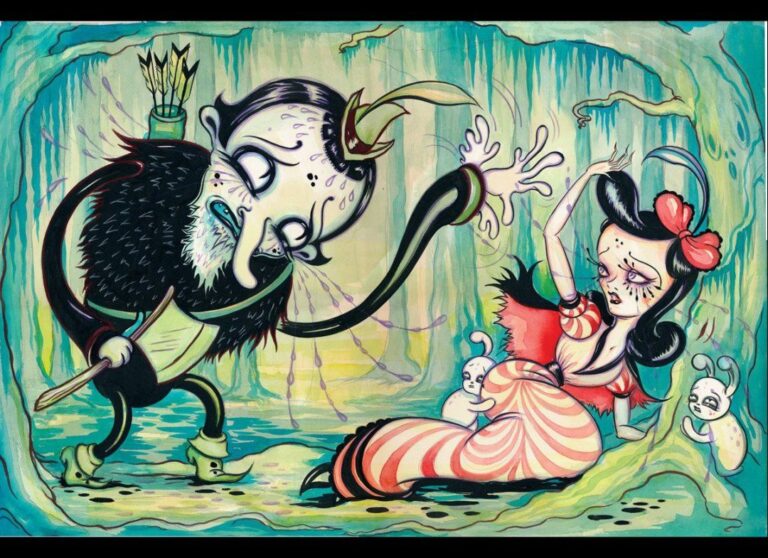The image is a stylized and fantastical drawing, portraying a scene reminiscent of Snow White and the Huntsman with an eerie, clown-like rockabilly twist. The scene is set within a dreary, blue-green forest that frames the characters. On the right, a distressed woman is shown kneeling on the ground in a red and white striped dress, her arm raised defensively. She has a larger-than-life head with black hair, drawing further attention to her anxiety. Surrounding her are two small, frightened rabbit-like creatures clutching onto her for protection.

On the left, the imposing figure of the Huntsman menacingly approaches. He is depicted with exaggerated features, including a long nose and multiple hands extending from one arm, adding to the surreal, creepy atmosphere. The Huntsman, dressed in a black and green fur coat, wears hunting boots and a plumed Robin Hood-style hat, and is equipped with a quiver of arrows on his back and a hatchet in his right hand. The tension in the scene is palpable as he waves his many-handed arm, possibly intending to strike, creating an unsettling and bizarre tableau.